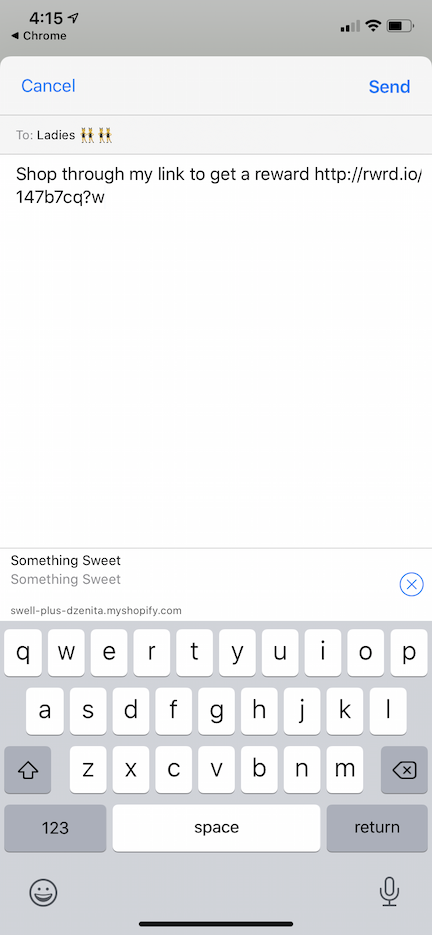A detailed and organized description of the mobile phone screenshot is as follows:

The screenshot captures a mobile phone interface, displaying various status indicators and an open email. At the top, there is a gray status bar showing the time as 4.15, along with an icon indicating that location sharing is enabled. Next to it, "Chrome" is displayed in black font, suggesting that the Chrome browser is open. To the right, there are icons representing a mobile signal with two out of four bars, Wi-Fi with full four bars, and a battery icon, which is half full.

Directly below the gray status bar, the email interface is visible. The email header features options in blue font: "Cancel" on the left and "Send" on the right. Addressed to "ladies," the email includes two emojis depicting standing ladies placed consecutively. The main body of the email contains a message written on a white background, which reads: "Shop through my link to get a reward." This is followed by a URL: http://rwrd.io/.147b7cq?w.

This detailed description elucidates the contents of the mobile phone screenshot, highlighting both the visual elements and textual information present in the email.